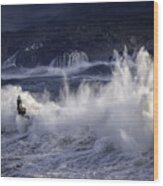The artwork depicts a very small, highly detailed painting that showcases a dramatic scene involving water and a person. In the center of the image, a massive wave crashes intensely, creating a towering splash of white foam that contrasts vividly with the surrounding dark blue water. To the left of this central splash, a black silhouette of a person appears to be engaged in water skiing or perhaps surfing, crouched down and gripping something in front of them, potentially being towed by a boat. The overall setting hints at a turbulent interaction between land and sea, with splashes suggesting water striking a rocky shore. The right edge of the image reveals the raw, brown wood of the canvas side, affirming the piece's painted medium. The background subtly includes elements like distant hills or house lights in the top left, enriching the scene with a hint of more tranquil surroundings beyond the chaotic foreground.